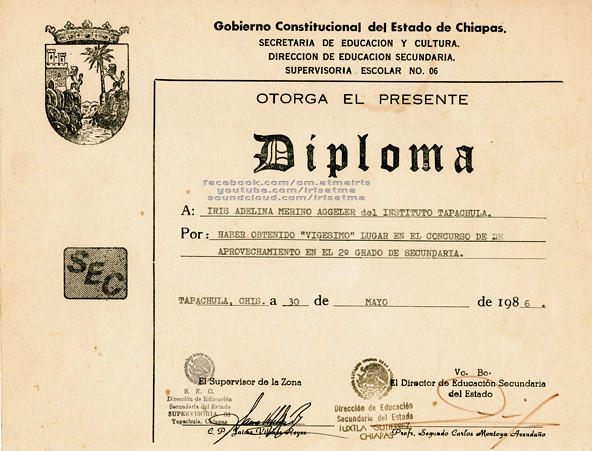The image depicts a very old-looking diploma, primarily in black and white, with text predominantly in Spanish. The document appears to be scanned and bears signs of significant aging, including yellowing and browning. At the top of the diploma, the header reads "Gobierno Constitucional de Estado de Chiapas, Secretaria de Educación y Cultura, Dirección de Educación Secundaria, Supervisoria Escolar número 06." Just below this text, the diploma declares in large, gothic script "Diploma."

Prominently featured on the top left corner is a crest, decorated with a crown and flanked by a pair of lions, with the abbreviation "SEC" visibly underneath it. The body of the document includes the phrase "Otorga El Presente Diploma," indicating the issuance of the diploma. While the diploma's specific recipient and purpose are not detailed by name in the description, the text corresponds to an award or certification dating back to 1986. At the bottom, the diploma is authenticated by two different stamps—one brownish and the other grayish—and signed by two individuals, verifying that the person met all necessary criteria.

Interestingly, despite the historical and official nature of the document, there are added details in a modern context, including digital additions such as addresses for Facebook, YouTube, and SoundCloud, indicative of perhaps a contemporary attempt at preservation or sharing in digital platforms.